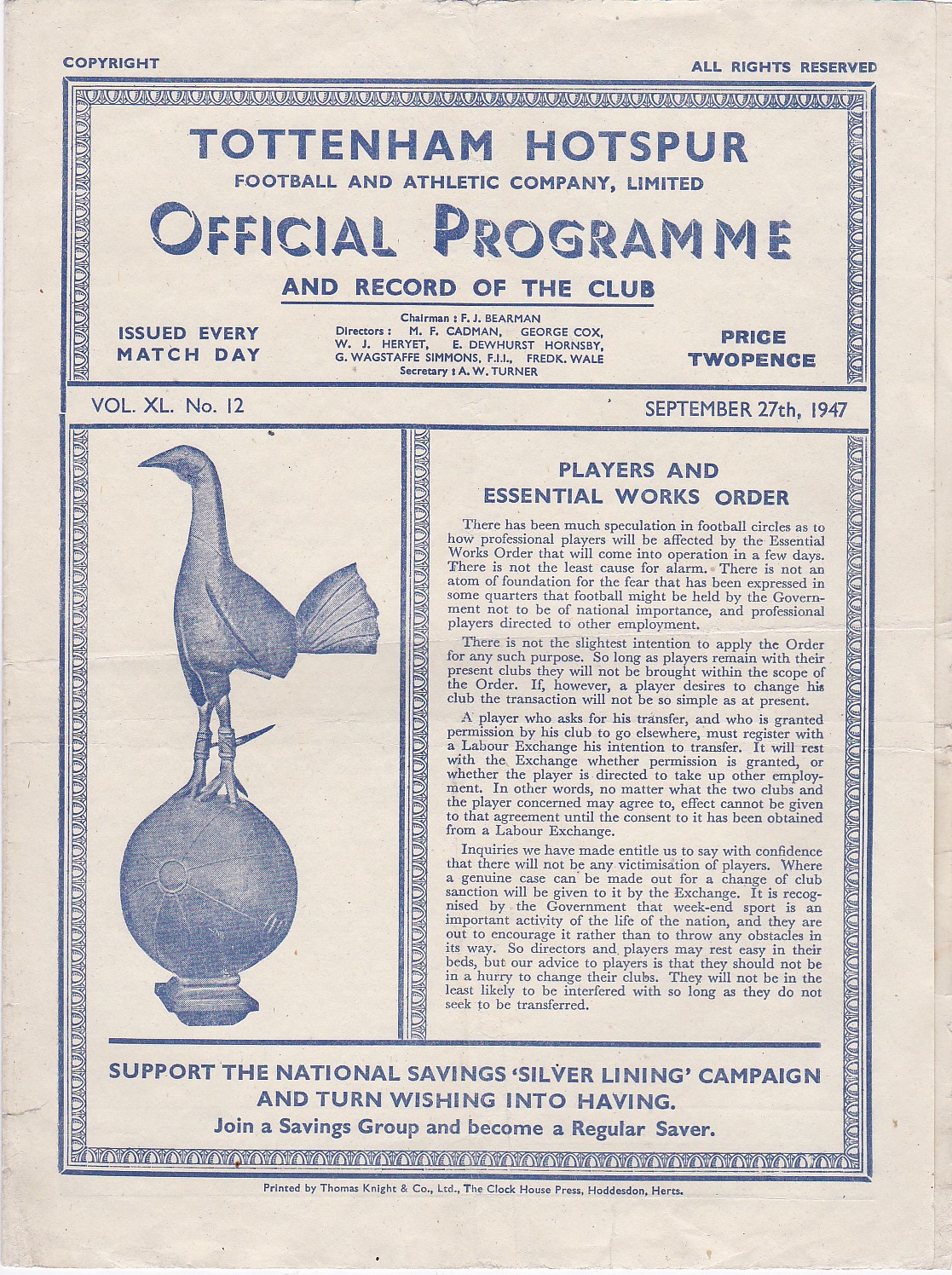The image depicts the cover of a vintage official football program for the Tottenham Hotspur Football and Athletic Company Limited, dated September 27, 1947. The background, initially white, has aged to a yellowish tint, while all text and illustrations are rendered in blue. At the very top, the heading announces it as the "Tottenham Hotspur Football and Athletic Company Limited Official Program and Record of the Club," issued on every match day, with a price of two pence. Below the heading, a series of names likely lists the club leadership. Dominating the center section, a notable illustration features a bird standing atop a spherical object resembling a globe, placed on a square base. To the right of this image is an article titled "Players and Essential Works Order," accompanied by substantial small print. Below, a promotional message encourages support for the "National Savings Silver Lining Campaign" with the slogan "turn wishing into having" and a call to join a savings group. The entire cover is framed with an intricate blue design. At the bottom, fine print notes the program was "printed by Thomas Knight and Company Limited" along with additional text not clearly legible.